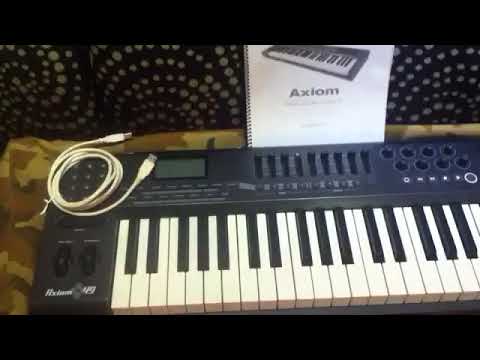The image depicts a horizontally rectangular keyboard with thick black borders at the top and bottom. The keyboard, likely an Axiom model as indicated by partially visible, blurred white lettering on the lower left side, features a coiled USB cable resting on its upper left side. The visible part of the keyboard showcases a mix of white and black keys, though the right side is truncated by the picture's edge. The keyboard rests on a camouflage-patterned fabric in green and brown, which is likely a sofa. Behind the keyboard, a patterned black wall or fabric with concentric white spiral polka dots is noticeable. A white booklet, assumed to be the keyboard's manual, stands vertically, displaying the brand name "Axiom" and an image of the keyboard on its cover. The keyboard also boasts various buttons, dials, and a digital display on the left side with additional control buttons beneath it.